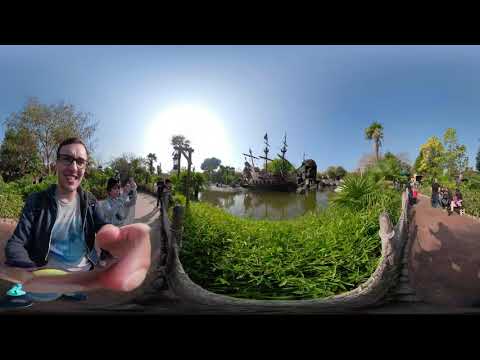In the image, an outdoor scene unfolds with a young man prominently positioned on the left-hand side. He has short, light brown hair, glasses, and wears a white t-shirt with a blue graphic, covered partially by a blue sweater and a gray jacket. The man is smiling and extending his arm out towards the camera, creating a visual distortion that makes his hand appear oversized. He stands on a brown pathway that curves semicircularly around the scene, branching into two sections.

Walking along the right-hand branch of the pathway are four or five people, including some families, adding a lively atmosphere. Behind the pathway, lush grassy areas and clusters of trees are visible. A wooden fence runs along the path's edge, preventing visitors from falling into a small pond with murky olive-green water. The pond houses an old-fashioned, shipwreck-like structure reminiscent of a scene from Pirates of the Caribbean, suggesting a themed attraction, possibly at a place like Disneyland. The background sky is a clear blue with the sun shining brightly, casting a warm light over the picturesque setting.